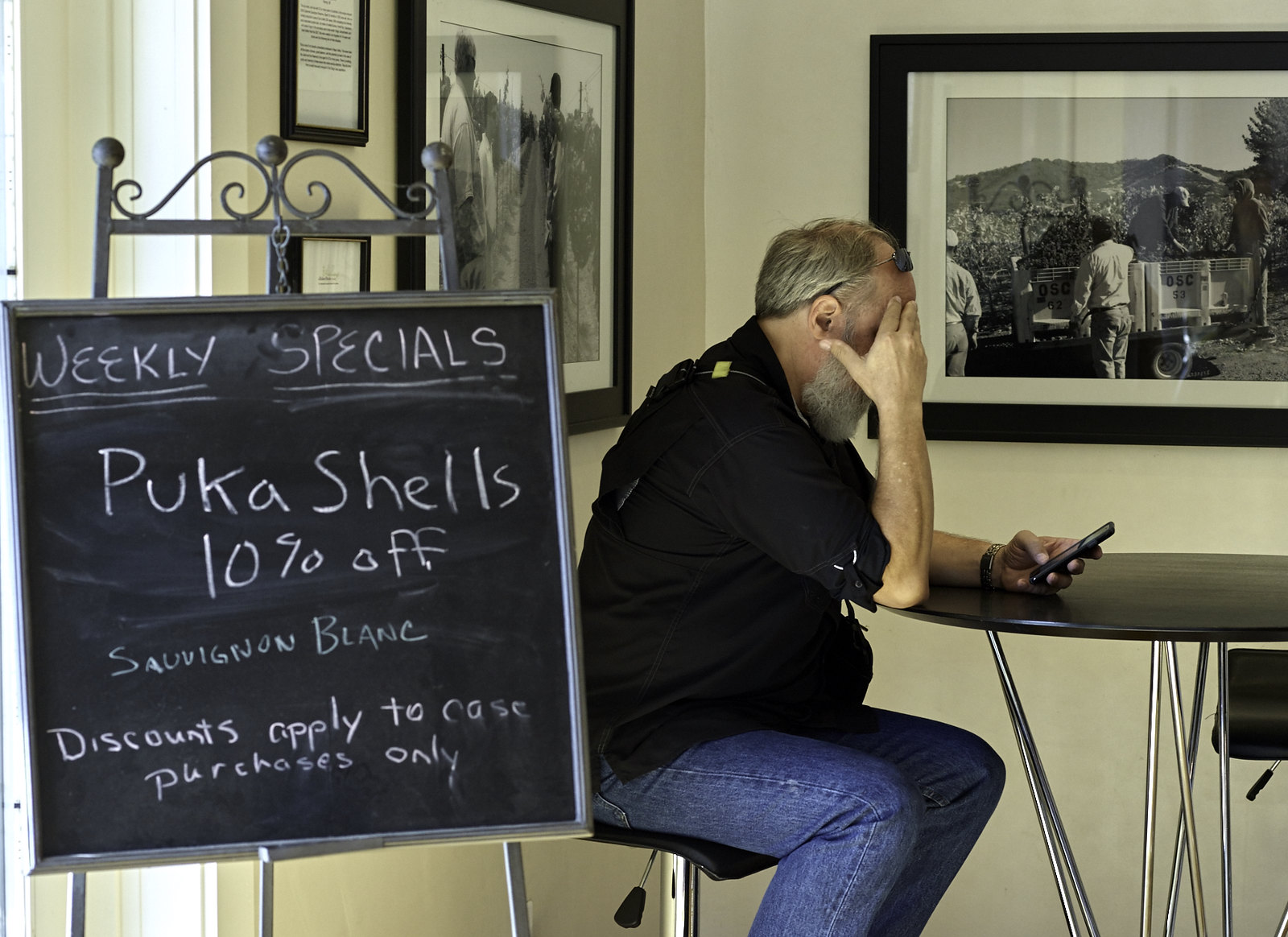In this detailed image, we see an older Caucasian male with a gray beard seated at a high-top black table with silver legs, sitting on an adjustable high-chair. He is wearing blue jeans and a black shirt. The man appears to be focused intently on his smartphone, holding his face in his hand, and his sunglasses are perched atop his head. He is situated in what appears to be a restaurant setting, indicated by the black chalkboard sign on the left side of the image that prominently displays "Weekly Specials" in white chalk, underlined twice. The specials listed include "Puka Shells 10% off," with additional text mentioning "Skagenegagwe block" and a discount that applies to case purchases only, with some parts of the text in green. The background features white walls adorned with two black-framed black-and-white photos, each with a white border. The overall atmosphere suggests a casual dining environment where the man is momentarily engrossed in his phone.